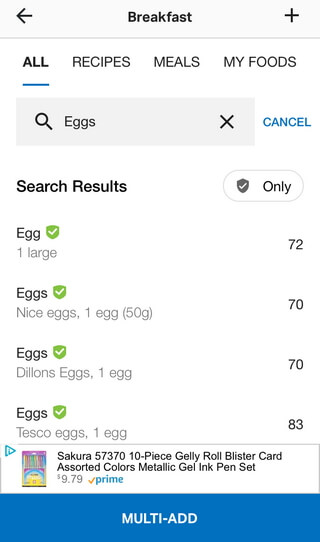A vertically oriented screenshot from the MyFitnessPal calorie tracking app is being displayed. The background of the app is white. At the top of the screen, there is a navigation bar labeled "Breakfast" in the middle. On the top left, there's a back arrow icon, and on the top right, there's a plus sign. Below this bar, there is a set of tabs: "All," "Recipes," "Meals," and "My Foods." The "All" tab is selected, evidenced by a blue underline and bold text.

Below the tabs, there is a light gray search bar, displaying a search for "eggs" with a magnifying glass icon on the left and an "X" on the right. To the right of the search bar, it says "Cancel." Beneath this, the screen shows search results for various egg entries, each featuring a green shield with a white check mark, indicating verified entries.

1. "Egg, one large" shows "72" calories to the right.
2. "Nice Eggs, one egg (50 grams)" details "70 calories."
3. "Dylan Eggs, one egg" is listed with "70 calories."
4. "Tesco Eggs, one egg" shows "83" calories.

At the bottom of the list, there is an advertisement for gel pens, detailing "Sakura 10-piece Jelly Roll Blister Card Assorted Colors Metallic Jelly Ink Pen Set" priced at "$9.79," accompanied by an Amazon Prime symbol. The very bottom of the screen features a blue banner with the text "More Ads" in white font.